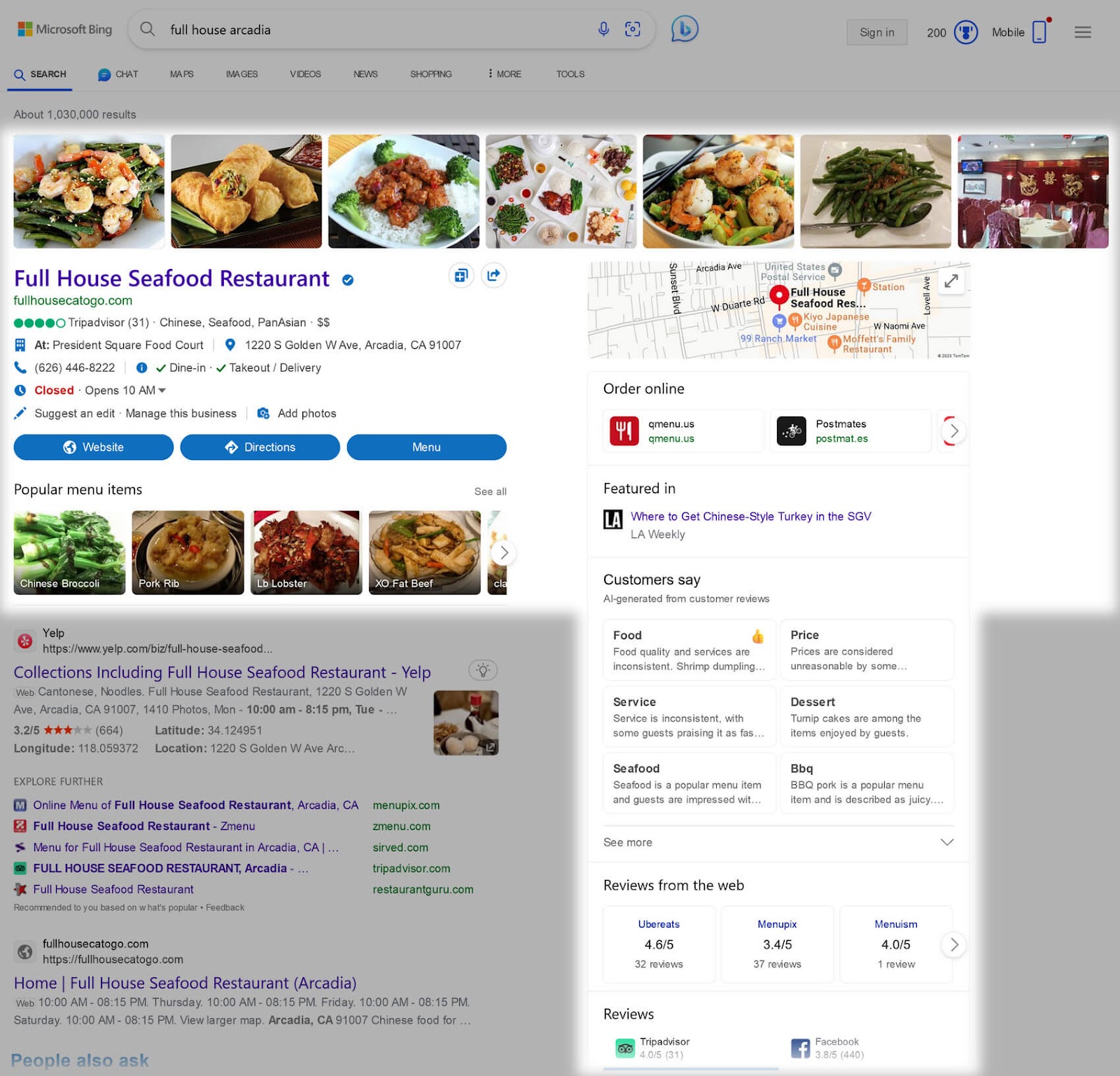Screenshot of a Microsoft Bing search results page for "Full House Seafood Restaurant." The page features the Microsoft logo on the top left and a search bar beside it, with options for signing in and mobile access. The majority of the page is grayed out, except for a highlighted section that resembles a "T" shape.

In the highlighted area, the restaurant's details are prominently displayed. This includes a series of photos showcasing dishes such as green beans with shrimp, egg rolls, and other Asian cuisine. Below the images, the restaurant has a four-star rating on TripAdvisor, accompanied by a map pinpointing its location. 

Additional information from other review sites such as Yelp is present, but less emphasized and shown in gray. The colored and detailed highlight draws special attention to the restaurant’s specific web page, while the remaining sections of the search results are subdued.